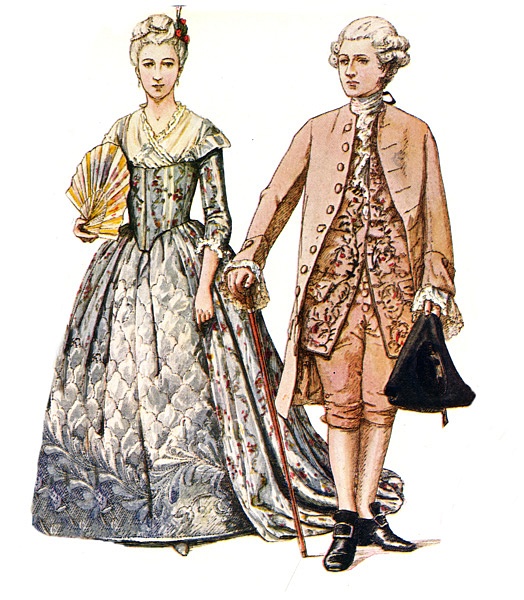This detailed image appears to be a colorful cartoon depiction of a man and a woman in formal, ornate attire reminiscent of the late 1700s. To the left, the woman is elegantly dressed in a stylish gown that blooms out at the bottom, featuring intricate frilly patterns in shades of gray and white. Her hair is elaborately styled, adorned with flowers, and she holds a fan in her right hand. Her dress has a cross-cut neckline and sleeves that extend just past the elbow, exposing her lower arms. 

On the right, the man is dressed in a peach-colored outfit, including a long overcoat and knickers, accentuated by a white high-necked blouse. He wears black shoes with silver buckles and holds a cane in his right hand while carrying a triangular Revolutionary War-style hat in his left. His hair is styled in white curls, reminiscent of George Washington. The overall scene reflects the formal and highly decorated fashion of the period, brought to life with vibrant colors and detailed patterns.